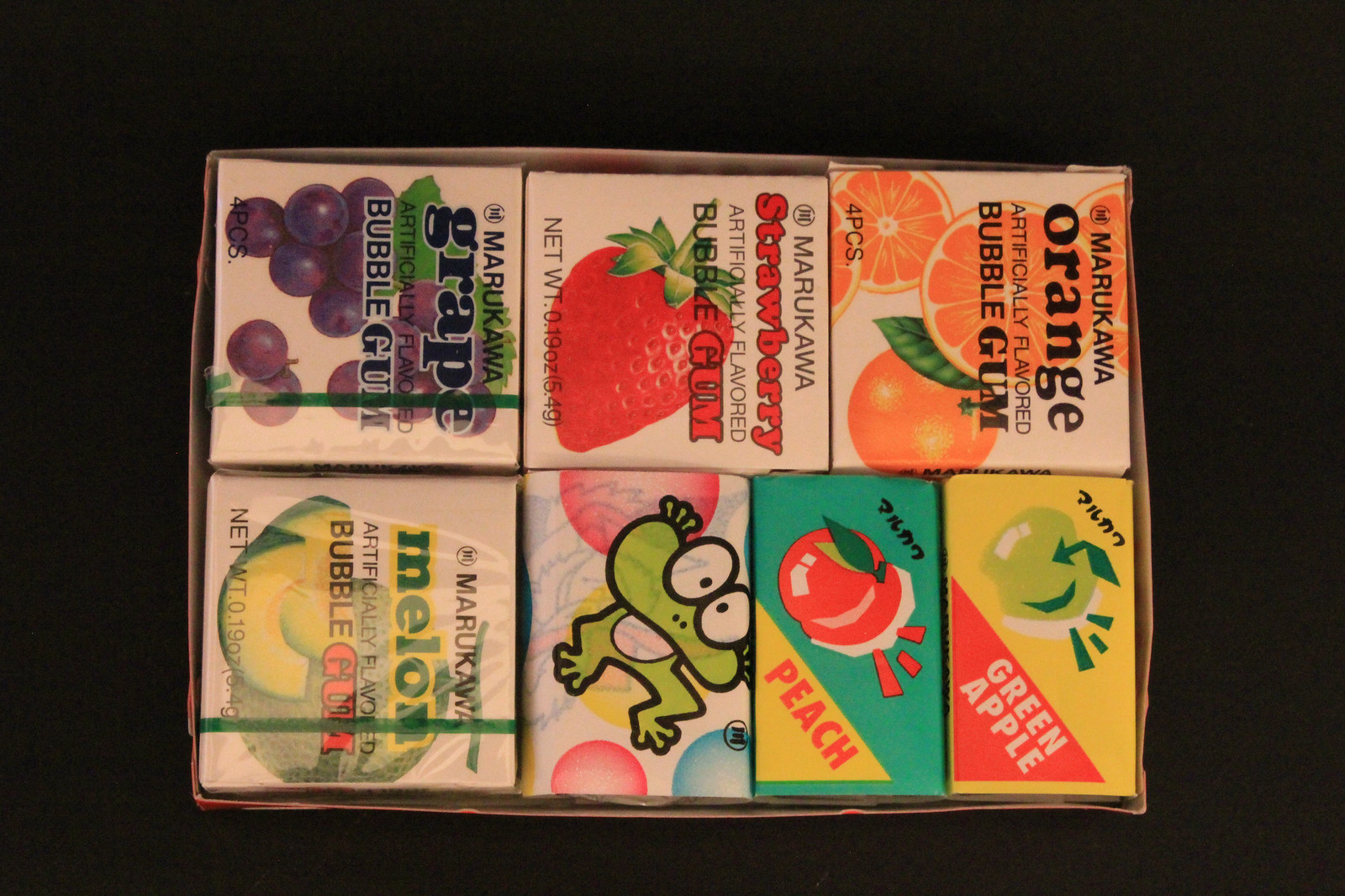This is a detailed top-down photograph showcasing a variety of Marukawa brand bubblegum packs arranged on a pitch-black background. Starting from the top left and moving downwards, there is an orange-flavored bubblegum pack displaying vibrant images of oranges and green leaves against a white background. To the left is a similar pack with strawberry-flavored gum, adorned with fresh strawberries. Adjacent to this is another pack featuring grape-flavored gum with images of tempting purple grapes.

Beneath the grape pack lies the melon-flavored bubblegum, still wrapped in its packaging and featuring melons. To its right, there's a distinctive pack wrapped in paper, embellished with a green cartoon frog and additional designs that remain somewhat obscure. Moving further right, there is a turquoise box labeled in Japanese and English as Marukawa peach-flavored gum, with a cute cartoon peach illustration. Finally, completing this collection is a yellow box labeled "Green Apple" both in Japanese and English, with a cartoony image of a green apple.

Each pack is neatly sealed, with some showing signs of plastic wrapping, and they are all aligned in a way that they face right, giving a clear view of the colorful and enticing designs meant to represent each flavor.